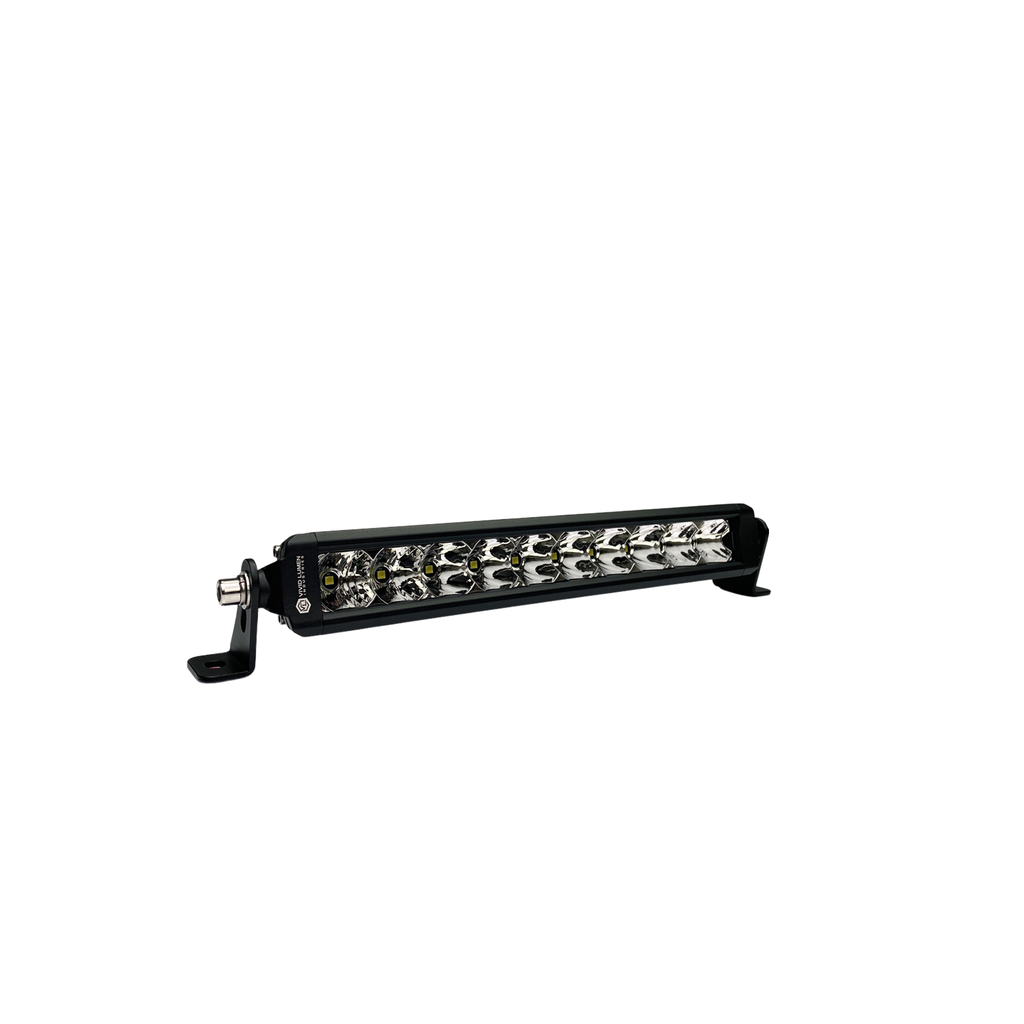This photograph showcases a sleek, black rectangular light bar designed for mounting on a sport utility vehicle or truck. The light bar is made of a durable material and features a sturdy foot on the left side with multiple holes for secure attachment. This foot ends in a shiny metal cap. In the center of the bar, there are several highly reflective circular lenses with small yellow dots in the middle, likely the bulbs, which are designed to shine brightly when the light bar is in use. Although some text or a logo is visible on the bar, it is too small to be legible.